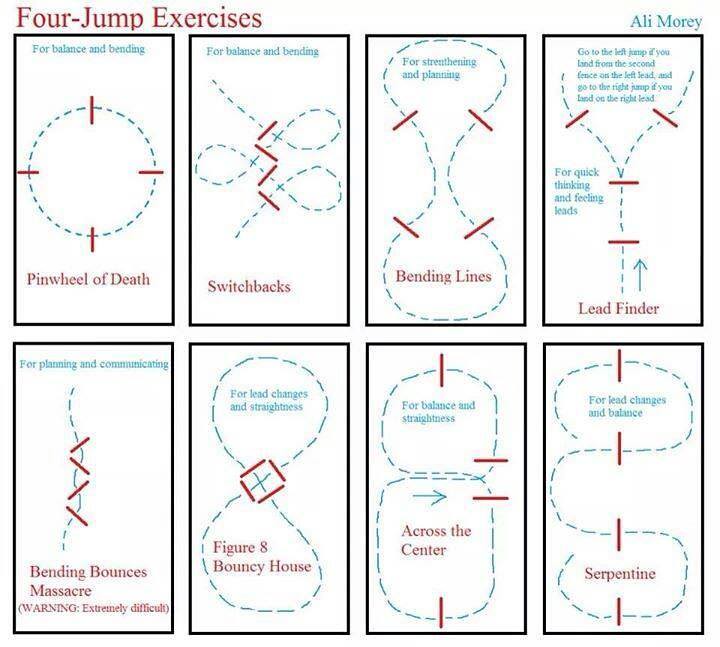The image is a set of instructional graphics titled "Four Jump Exercises" by Ali Mori, displayed in eight rectangular panels arranged in a 4x2 grid. The title "Four Jump Exercises" is displayed in the top left corner in brown text, with Ali Mori's name to the right in green. Each panel highlights different exercises and concepts for dance or gymnastics.

1. **Pinwheel of Death:** The first panel, labeled "For Balance and Bending," features a dotted circle with red lines at the top, bottom, left, and right positions. It is titled "Pinwheel of Death."

2. **Switchbacks:** The second panel emphasizes "For Balance and Bending" again but showcases a swirling figure-eight pattern dotted in blue with a red sideways "W" line, under the title "Switchbacks."

3. **Bending Lines:** The third panel is intended "For Strengthening and Planning," visualized through an hourglass shape made up of bending red lines forming a diamond-like pattern.

4. **Lead Finder:** The fourth panel provides guidance "For Quick Thinking and Feeling Leads," showing a blue dotted Y-shaped line with instructions for landing on left or right leads. Titled "Lead Finder," it includes red lines before and after the Y's fork.

5. **Bending Bounces Massacre:** The fifth panel, labeled "For Planning and Communicating," displays a curved blue line and a sideways "W" red line, accompanied by a warning: "Bending Bounces Massacre - Extremely Difficult."

6. **Figure Eight Bouncy House:** The sixth panel, "For Lead Changes and Straightness," features a blue dotted figure-eight with a central red diamond shape made from four lines, labeled "Figure Eight Bouncy House."

7. **Across the Center:** The seventh panel, which does not specify a purpose, shows a blue arrow crossing the center of four red lines, positioned in a unique arrangement.

8. **Serpentine:** The final eighth panel, titled "Serpentine," aims "For Lead Changes and Balance" and is illustrated with an S-shaped blue curve and four vertical red lines.

Each panel mixes visual elements with instructional text to guide users through a series of structured exercises aimed at improving different aspects of physical training.